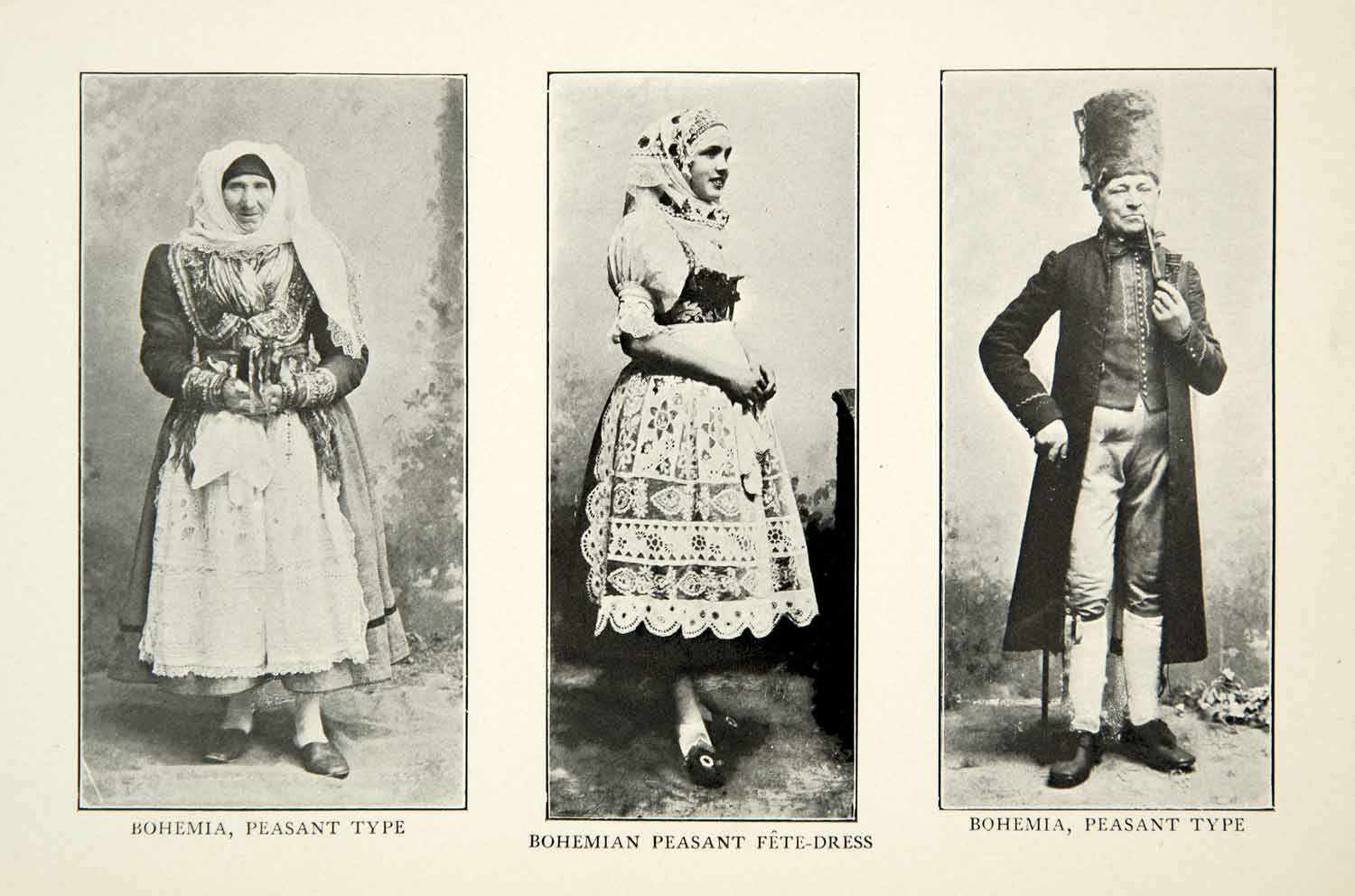This image features a photograph of a yellowed page divided into three rectangles, each holding a black and white photograph of individuals in traditional Bohemian attire from an older time period. 

On the far left, the photograph depicts an older woman labeled "Bohemian peasant type." She is dressed in a long, baggy garment with a white head shawl over black fabric, layered with a frilled white petticoat and apron. Her long-sleeved dress features puffy sleeves, and she wears simple flat shoes with stockings. The woman’s hands are held out in front of her waist, adding to the authenticity of her peasant attire.

The middle photograph, labeled "Bohemian peasant fete dress," shows a younger woman, possibly a teenager, standing in profile while facing right. Her ornate dress consists of a headdress with decorative patterns, a laced and puffy white apron, and embellished flat shoes adorned with a medallion on the toe. The long sleeves of her dress are puffy at the shoulders and wide at the ends, bestowing a festive, celebratory air to the ensemble.

On the far right is an image labeled "Bohemian peasant type," depicting a man dressed in traditional male attire. He wears a tall fur hat and smokes a pipe that touches his lips. His outfit includes a long overcoat extending to his calves, a buttoned vest underneath, long pants, white socks, and dark shoes. He holds a walking cane, adding a touch of distinction to his peasant look.

All three photographs are black and white, printed on vanilla-colored paper, enhancing the antique feel of this descriptive representation of Bohemian peasant fashion.